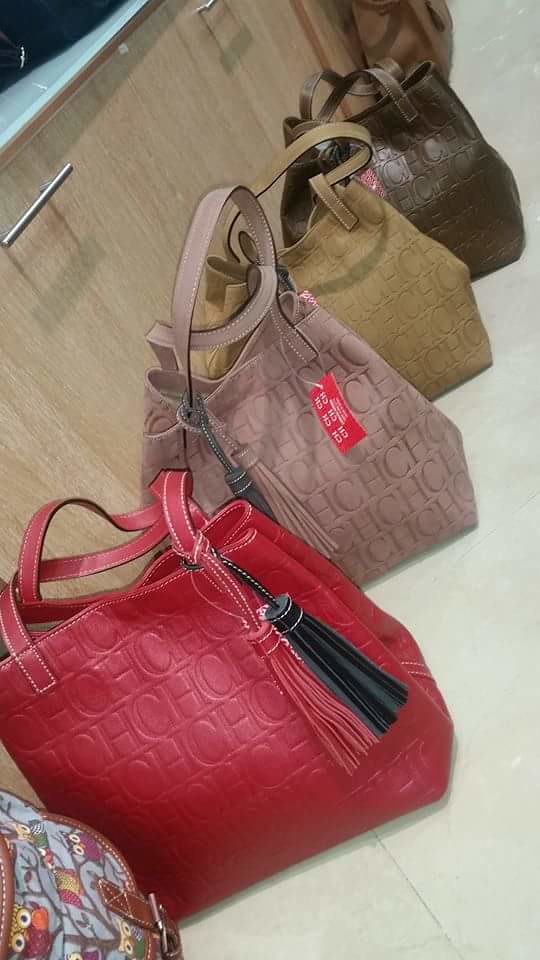The image showcases a room featuring a floor-to-ceiling view of several handbags lined up in front of a light brown cabinet with silver horizontal handles, set against a polished, light-colored tile floor. The bottom left corner presents a reddish-brown leather purse adorned with whimsical illustrations of owls perched in a tree, complete with a silver clasp. To its right sits a red leather purse with red and black tassels and white stitching, adorned with "CH" initials. Following this, there are three more handbags, each with "CH" initials: a light brown one, a tannish-green one, and a dark brown one, all similar in brand but differing in color. Lastly, at the top of the arrangement is a lighter, almost reddish-brown handbag that lacks the "CH" initials, completing the display of six handbags in total.